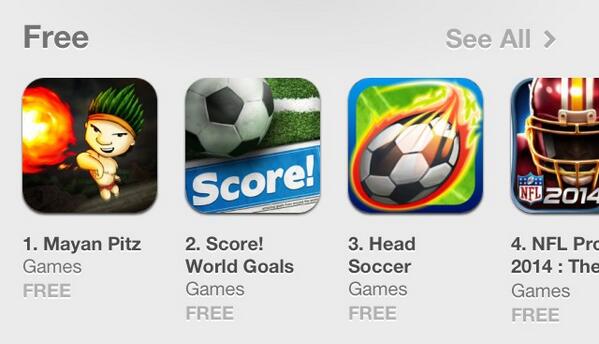This image depicts a screenshot of an older version of the Google Play Store, specifically from the section for free games. There's a clear numerical listing of four games, each accompanied by its respective cover image and title. The games are shown as follows:

1. **Mayan Pits**: The cover features a male character throwing a red fireball.
2. **Score World Goals**: Displayed with an image of a soccer ball and the word "Score" beneath it.
3. **Head Soccer**: Illustrated with a soccer ball engulfed in flames.
4. **NFL Game**: Partially visible title, but shows an NFL player in a helmet facing the viewer.

At the top left corner, a label indicates that these games are categorized as free. In the top right corner, there's an option to see all games in this category.